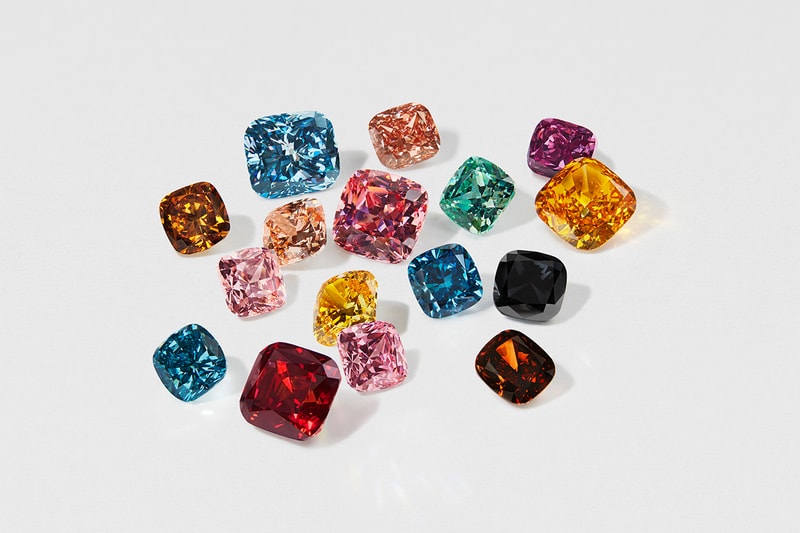This high-resolution photograph showcases approximately 20 professionally cut gemstones arranged against a light gray background. The gemstones are framed in the center, displaying a vibrant array of colors including blue, dark red (likely a ruby), pink, orange, yellow, and black. Each gem has a unique square or rectangular shape with multiple facets, reflecting a spectrum of hues and adding depth to their appearance. The precision cutting and professional lighting highlight their reflections without any distracting glare, emphasizing each gemstone's clarity and brilliance in what appears to be a meticulously staged product photo.